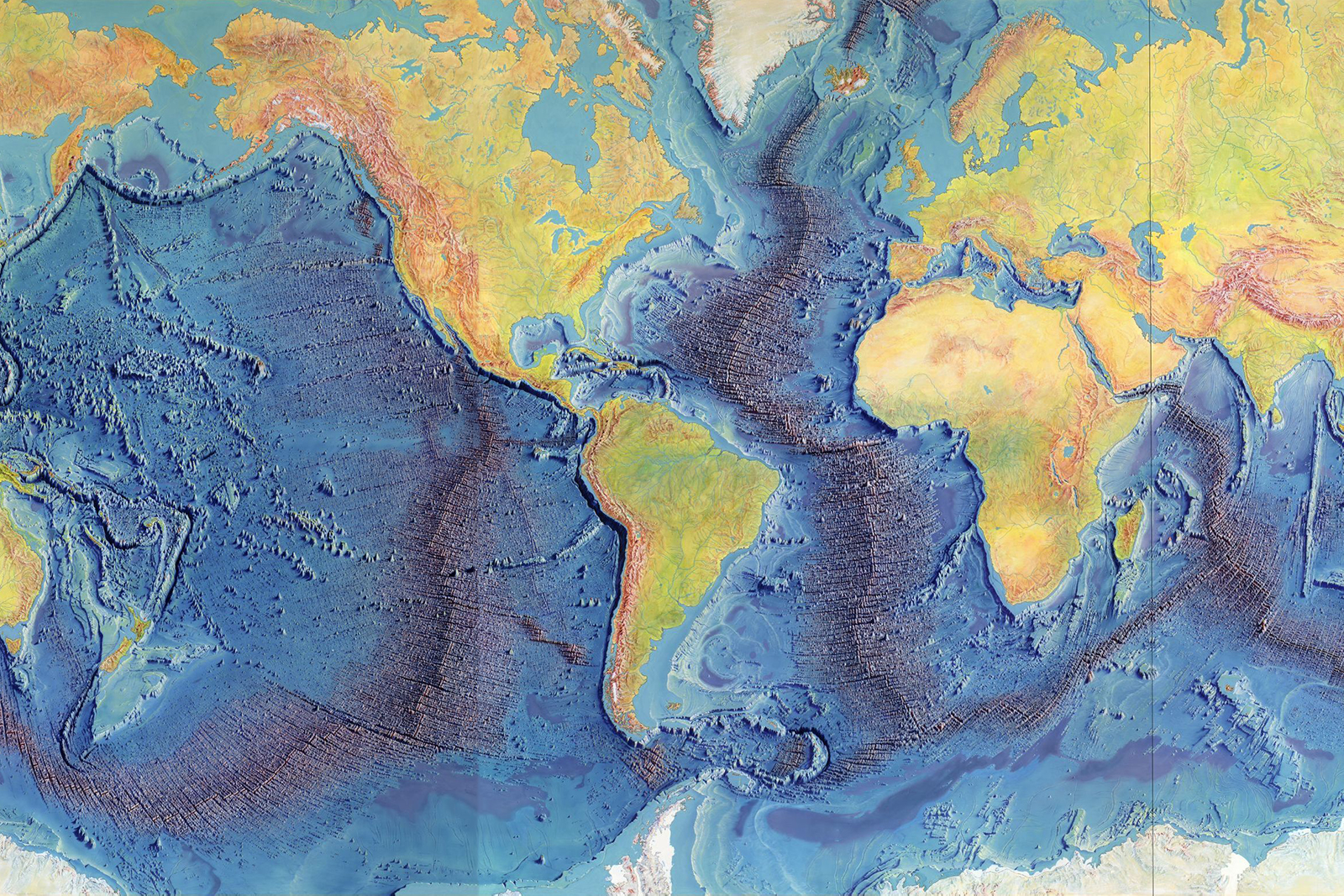This landscape-oriented color photograph showcases an intricately detailed 3D relief map of the world, highlighting both terrestrial and oceanic features. The continents are vividly depicted in a yellowish-green hue with reddish-brown regions indicating higher mountain ranges. In contrast, ocean depths are illustrated using a gradient of blues, with lighter blue signifying shallower continental shelves and deeper blue indicating the abyssal regions. The deepest ocean trenches are rendered in purple, adding a striking contrast. White areas mark the frozen continents, prominently at the center top and bottom of the map. Notable geographic details include the majority of the Pacific and Atlantic Oceans, with Southeast Asia and the top of Russia notably cropped out. This topographical map offers a comprehensive elevation and depth portrayal, utilizing varied colors to denote different heights and depths across the globe.